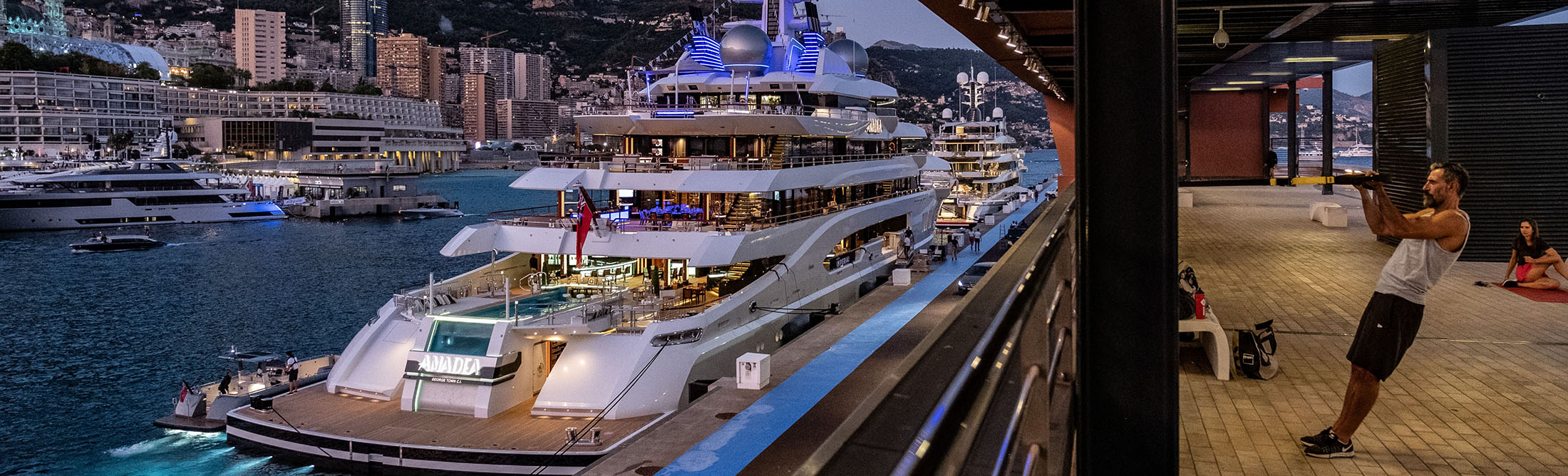This horizontally rectangular photograph consists of two distinct sections, divided by a vertical black line. The left side of the image features an outdoor nighttime scene showcasing a luxurious, multi-story yacht illuminated with amber-yellow lights, and adorned with wooden decks and satellite dishes. The yacht, clearly belonging to a wealthy individual, is docked along a cement pier with additional yachts visible against a distant city skyline of tall high-rise buildings atop a hill. This side is bathed in shades of gray, blue, and tan, enhancing the natural and artificial lighting effects over the water and the vessels.

The right side of the image transitions indoors to a gym setting with gray brick flooring, also captured under artificial light. A man in shorts and a t-shirt is engaged in a wall exercise, pulling on yellow resistance bands attached to a wall hook. Positioned in the background, near the center-right, a woman stretches on a yoga mat. This indoor segment contains elements of black, gray, and neon blue, subtly blending with the overall ambiance of the nighttime scene outside.

Together, the composite image creates a stark yet captivating juxtaposition of an opulent outdoor marina with a serene indoor gym, separated yet harmoniously blending through the seamless split of the photograph.